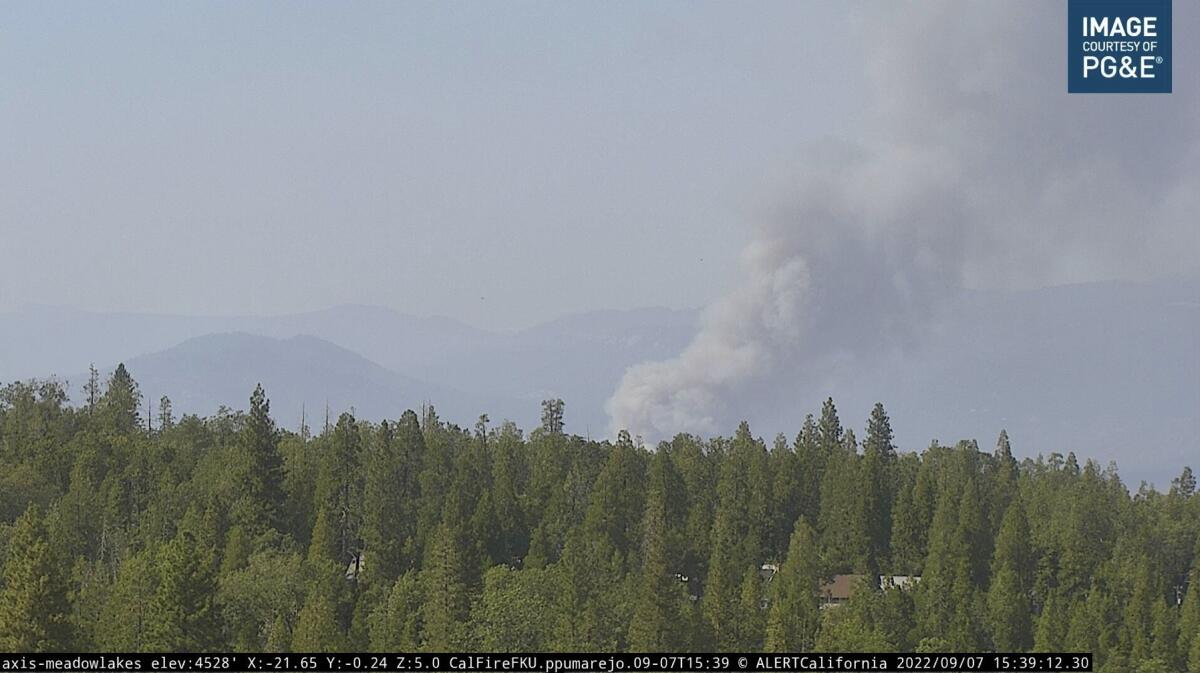The image appears to be a photograph captured possibly from a news broadcast or observation camera, showing a forest fire in a wooded area. In the foreground, a tree line with a mix of tall pine trees and deciduous trees frames the scene, while glimpses of house roofs can be seen nestled among the trees. The background features a hilly terrain obscured by a significant plume of white smoke, billowing from the center of the frame and drifting towards the right. The smoke casts a hazy veil over the sky, rendering it void of its usual blue and giving the distant hills a grayish hue. At the top right corner, a blue square with white letters reads "Image courtesy of PG&E." At the bottom of the image, a black bar with white text provides detailed information, including "Access Metal Lakes, elevation 4528 feet, Cal Fire, Alert California," along with more precise coordinates and a timestamp.